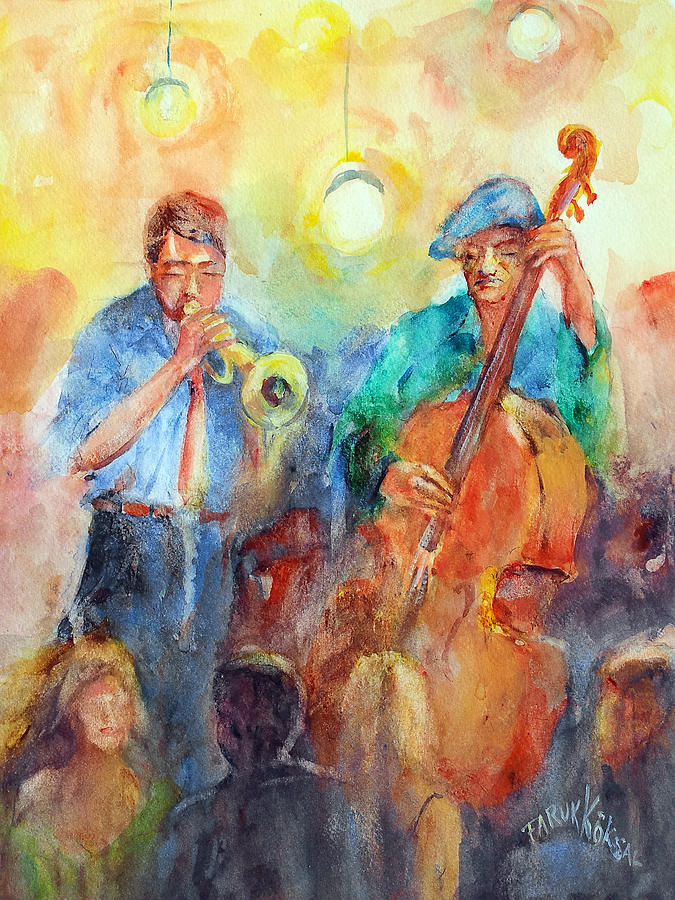This painting captures a lively musical scene set in a club, characterized by an impressionist style with rough, sketchy details that evoke a sense of movement and energy. Dominating the composition are two musicians: a trumpet player with short brown hair, eyes closed in concentration, wearing a blue button-up shirt, an orange tie (sometimes perceived as red), and blue jeans. He holds a golden trumpet to his lips, passionately blowing into it. To his right, a cellist dressed in a green jacket and a light blue artist cap (sometimes described as a blue shirt and blue cap) plucks at the strings of a large burnt-orange cello. The background is filled with swirling hues of yellow and orange, giving the impression of a vibrant, dynamic atmosphere, and includes two yellowish orbs that resemble light bulbs or lights hanging from the ceiling. 

In the foreground, below the musicians, a small crowd is gathered, possibly dancing or seated. The crowd includes a woman in a green dress with long blonde hair, a man in a dark jacket with his back turned, another woman with blonde hair just visible, and the face of an additional gentleman on the far right. The painting exudes an impressionist aura with its textured, almost faded look, and is signed "Farooq Kokasal" in the bottom right corner.